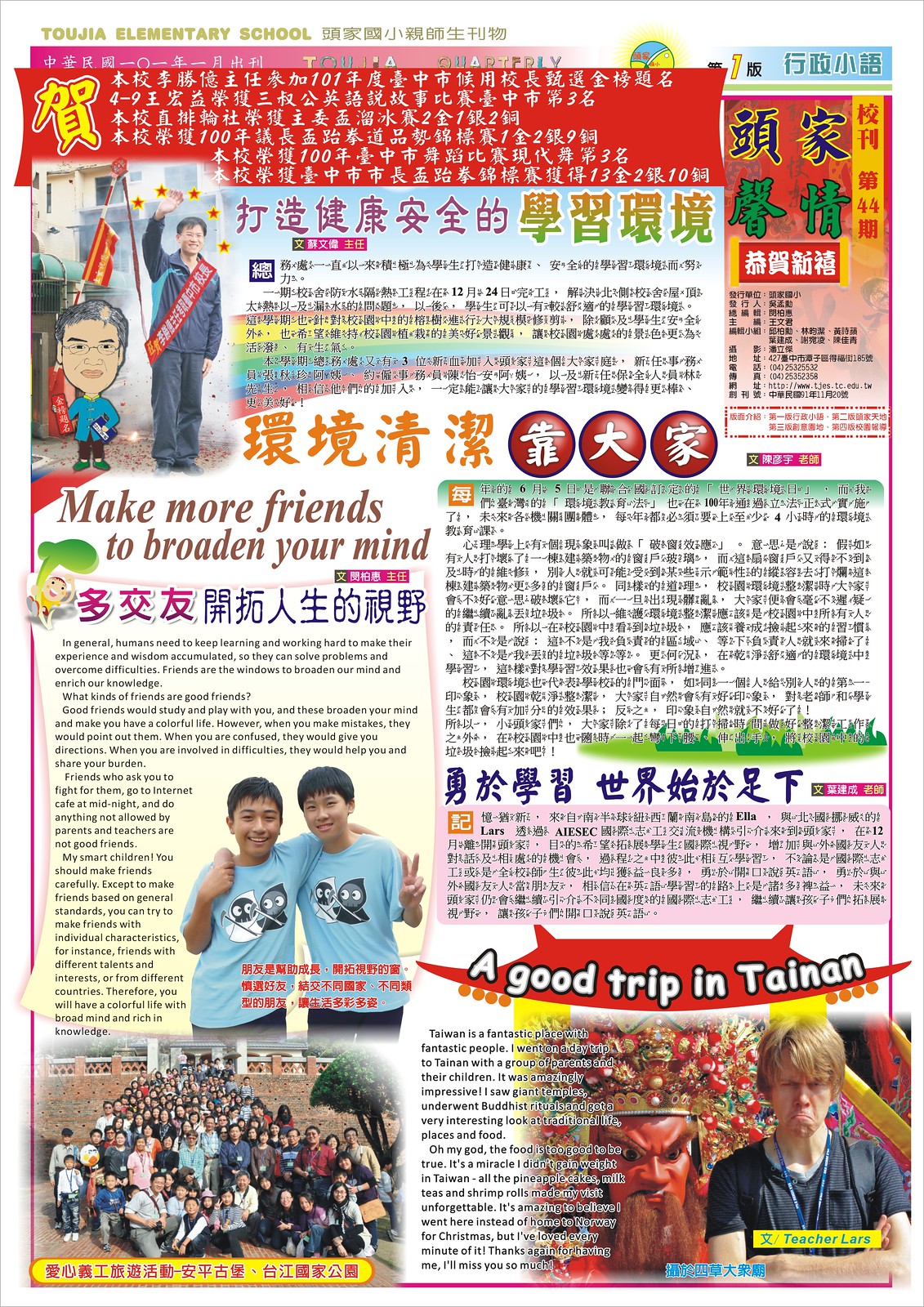The image is a vibrant, rectangular advertisement calendar predominantly in Chinese with some English elements. The calendar's header features “Tujia Elementary School” in English on a white border, followed by an assortment of colorful Chinese characters, including bold yellow, red, and rainbow-colored ones. A man in a grey tracksuit, adorned with a red sash and waving, is pictured at the top alongside a cartoon figure with an oversized head. Below, an English headline reads, “Make More Friends to Broaden Your Mind,” surrounded by diverse graphics, pink and black Chinese characters, and more text in black. 

In the middle-left section, a photo captures two boys in matching blue t-shirts featuring cartoon designs, with their arms around each other; one of them is holding up a peace sign. Beneath this image, a group photo shows people lined up and posing.

On the bottom right, a section titled, “A Good Trip to Tainan,” showcases a white man with a frowning face, identified as Teacher Lars. He is placed next to a statue of a red-faced, bearded king, possibly imitating the statue’s expression. The overall layout appears busy with a mix of pictures, titles, and diverse graphics, creating a lively and somewhat chaotic visual presentation.